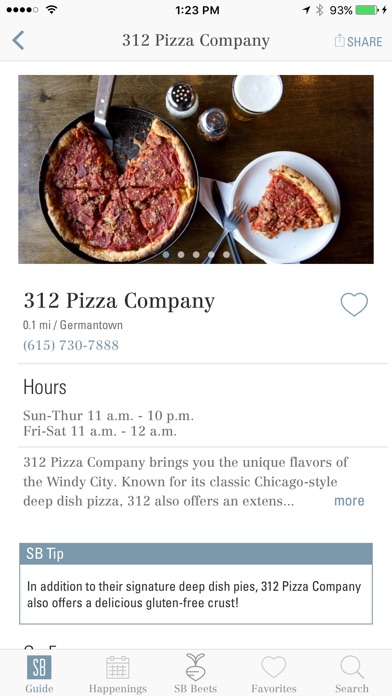Here's a cleaned-up and detailed caption for the image described:

---

A screenshot of the 312 Pizza Company website viewed on a mobile phone. The top of the screen displays the status bar with three horizontal lines on the left, the current time (1:23 p.m.) in the center, and an arrow next to a 93% battery indicator on the right. Below, there's a navigation bar with a back arrow on the left, "312 Pizza Company" centered in gray text, and a share icon on the right.

The main content features an appetizing photo of a whole pizza alongside a slice placed on a white plate with a fork, surrounded by salt, pepper, and other condiments on a brown table. Below the image, "312 Pizza Company" is prominently displayed, followed by a heart icon, a distance of "0.1 miles," and the location "Germantown." The contact phone number, 615-730-7888, is highlighted in light blue text.

A gray bar indicates the restaurant's hours: "Sunday to Thursday, 11 a.m. to 10 p.m." and "Friday to Saturday, 11 a.m. to 12 a.m." Following the hours is a brief description: "312 Pizza Company brings you the unique flavors of the Windy City, known for its classic Chicago-style deep dish pizza. 312 also offers... More."

At the bottom, a bluish-gray bar features an "SB Tip" in white text with a box containing information: "In addition to their signature deep dish pies, 312 Pizza Company also offers a delicious gluten-free crust." 

The final navigation bar includes options from left to right: "SB Guide," "Happenings," "SB Beats," "Favorite," and "Search."

---